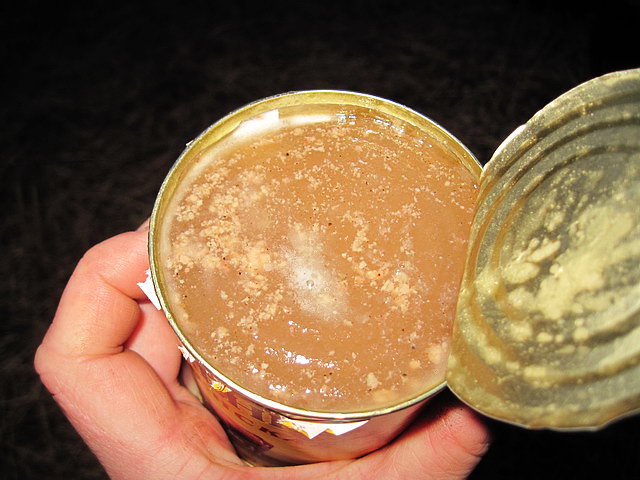In the image, a can of food is held by a person's hand against a solid black background. The can has been opened, with the lid still attached on one side, revealing a gooey, light brown substance inside, which appears gel-like or possibly soupy. The food inside shows indents from the lid, with concentric circles that get smaller towards the center. Speckles of mold or white foam are visible on the surface, indicating some spoilage. The can's label is torn and partially visible but unreadable due to the angle. The can, jaggedly cut, shows traces of the food and some lighter crumbles stuck to the lid. The hand holding the can reveals the thumb, middle, and ring fingers, suggesting a careful grasp due to the potentially sharp edges.